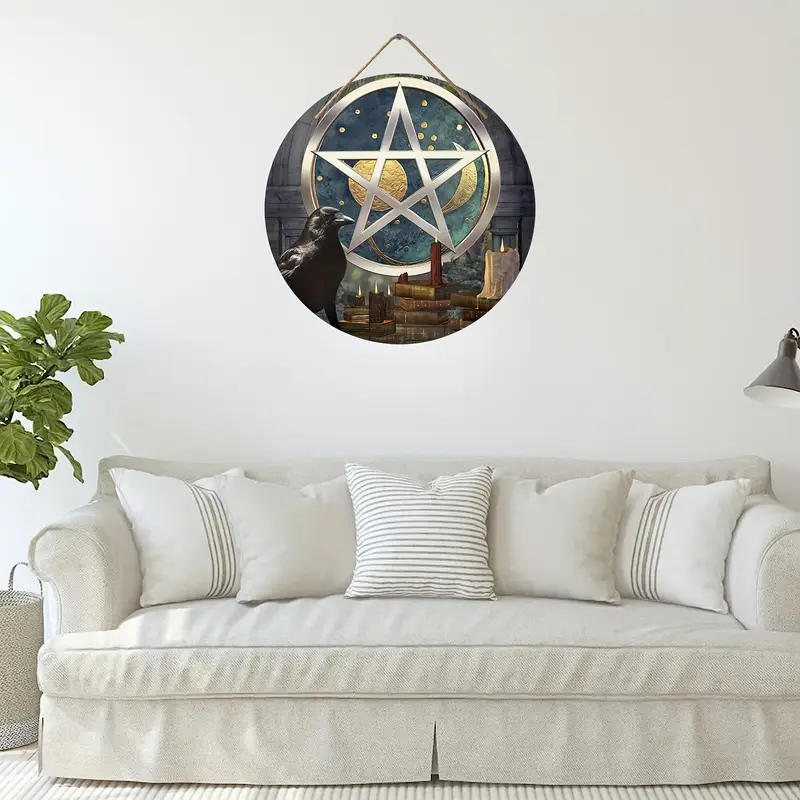This photograph captures a richly detailed living room scene that evokes a sense of mystique and enchantment. Central to the image is a white sofa adorned with five throw pillows, each featuring decorative stripes, some vertical and some horizontal, adding a subtle texture to the setup. The couch appears to have an apron running along its bottom, seamlessly blending with the room's sophisticated aesthetic. To the left of the sofa, a lush indoor plant in a light-colored basket enhances the room's natural feel, while on the right, a reading lamp peeks into view with only its shade visible.

Dominating the wall above the sofa is a striking circular wall hanging, suspended by a piece of rope. This artwork showcases a silver pentagram enclosed within a circle, set against a dramatic celestial backdrop depicting the sun, the moon, and myriad stars, conveying a sense of space and mystery. Below the painting in the foreground, a candle and a raven figurine rest on a surface, accompanied by a few books, reinforcing the magical and somewhat occult ambiance of the room. The background, painted in dark tones, adds to the room’s foreboding and captivating atmosphere. The setting is completed with a white carpet featuring subtle linear patterns, grounding the overall composition of this intriguing and mystical living room.